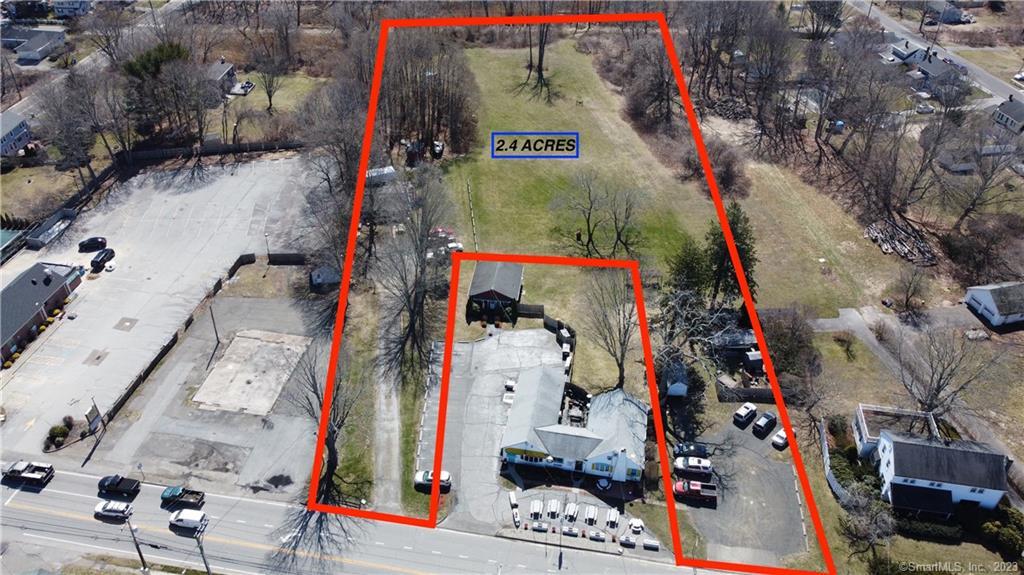This image, seemingly taken by a drone for real estate purposes, showcases a residential area with distinctive features. In the landscape-oriented photo, at the very bottom center, there is a prominent building consisting of two connected structures with a courtyard in the back. Surrounding this central building, a large parking lot is situated on the right, accompanied by picnic tables in the front, fenced off from a smaller house behind it. 

Residential streets frame the top left and top right corners, characterized by gray and white houses, and a mix of gray and black rooftops. The greenery in the area features broad acres of vibrant green grass dotted with trees, most of which are bare, with brown or gray stems and branches, and some retaining green leaves. 

Several parking lots can be observed: one on the left side with light gray pavement hosting a couple of black cars, and another on the right containing a dark gray lot with three white cars and a gray car alongside a red truck. In the middle of the image, a gray building with a white rooftop stands adjacent to a house with a gray and black rooftop.

Prominent in the photo is a red property boundary line that encloses the significant structures and the expansive field behind them. Inside this boundary, labeled in black letters within a blue rectangle, there is a notation of "2.4 acres". Further in the background, a mixture of wooded areas and additional houses and businesses round out this vibrant snapshot of the community.